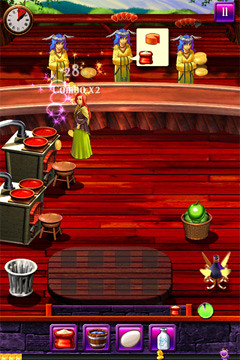This screen capture, depicted in vertical orientation likely indicating it's from a mobile game, showcases a dynamic scene set on a rich red hardwood floor. At the top-left corner of the screen, there is a white clock with a red section, suggesting a timer for the gameplay, complemented by a pause button in the top-right corner. Central to the scene are three women standing behind a broad wooden countertop, dressed in long yellow tops and green dresses with striking blue hair, resembling princesses with angel-like wings emerging from their heads.

In the foreground, next to two green ovens, each with two red pots possibly containing soup, stands a young woman adorned in a yellow and blue top, a green dress, and with flowing red hair, surrounded by a shimmer of white sparkles. Below her, a basket brimming with green apples sits on the deck. The ovens appear to be attached to pipes that extend off-screen, suggestive of a detailed and elaborate kitchen setup.

Adjacent to the ovens, a small round wooden stool is positioned, and next to it, a metal trash can is visible. Further down, on a purple brick lower section of the screen, various icons—representing flour, a water bucket, an egg, and a milk bottle—are arrayed, part of a menu or inventory system critical to the game's mechanics. The overall ambiance blends elements of fantasy and domesticity, marked by attention to detailed costumes and animated elements.